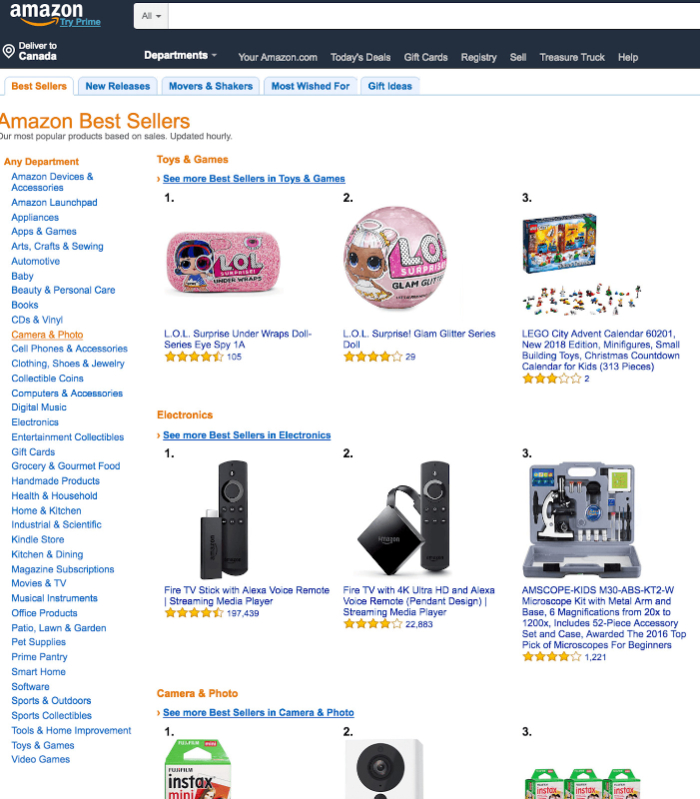The image displays the Amazon.ca homepage, indicating it is the Canadian version of Amazon. In the top left corner, the well-known Amazon logo is prominently presented, with "Try Prime" written in blue text and underlined just below it. Beneath the logo is the phrase "Deliver to Canada," confirming the geographic focus of the web page.

At the top center, there's a large, empty search bar with the word "All" at its leftmost end, signifying that searches can be conducted across all departments. Below this search bar is a horizontal menu featuring various categories: "Departments," "You are on Amazon.com," "Today's Deals," "Gift Cards," "Registry," "Sell," "Treasure Truck," and "Help."

Lower down the page, additional clickable categories are listed vertically on the left side: "Bestsellers" (highlighted in orange text), "New Releases," "Movers and Shakers," "Most Wished For," and "Gift Ideas," all in blue text. 

At the center of the image are product listings from Amazon. Featured prominently at the top is the "Toys and Games" section. Below this, one specific item is highlighted: a "Surprise Under Wraps Doll Stories" toy. To the right of this toy, there is a "Lego City Advent Calendar," showcasing available holiday-themed items.